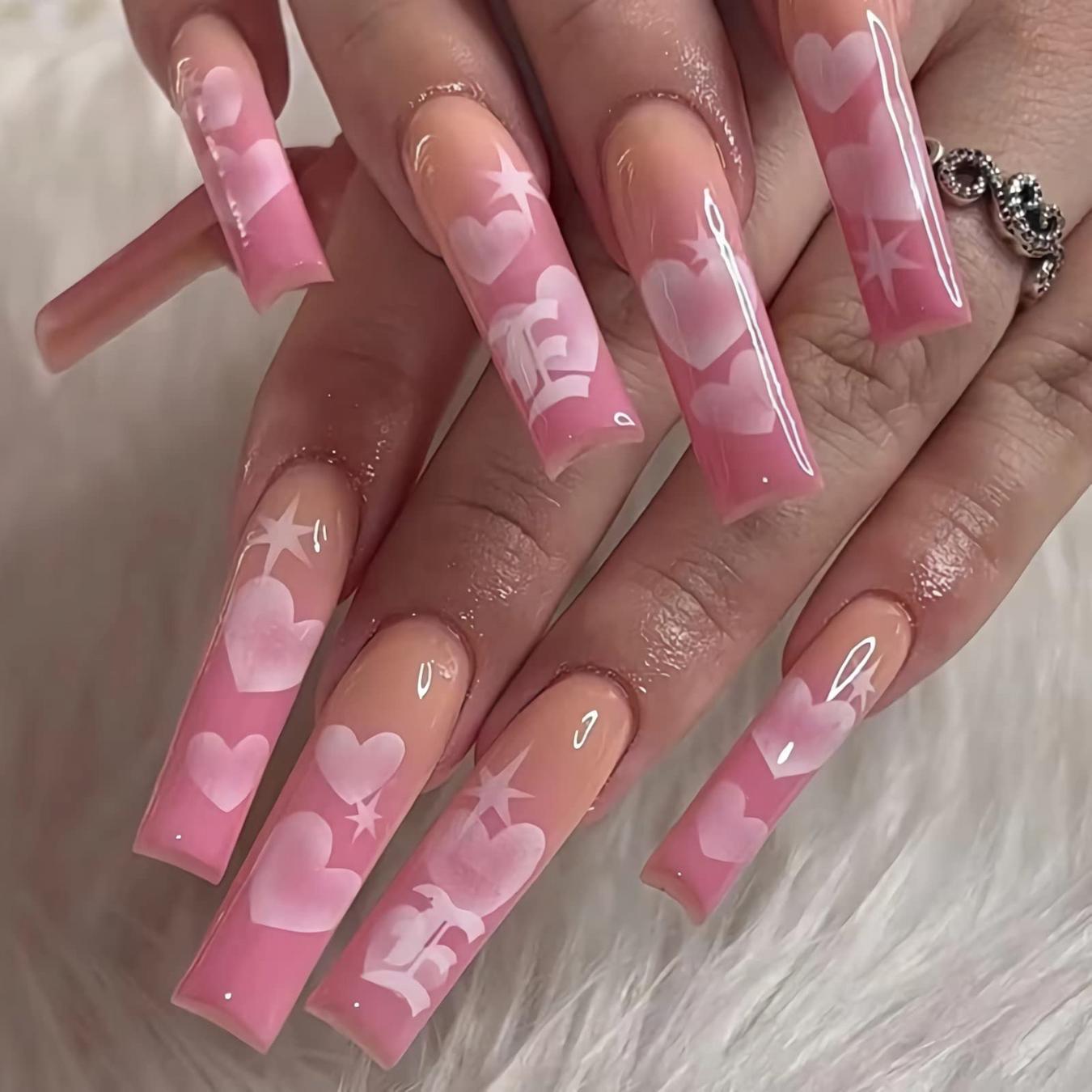The image depicts a woman with fair skin showcasing her freshly done, extremely long, glossy nails, posed against a backdrop of soft, white fur, which could be a furry blanket or resembling dog fur. The nails are notably elongated, squared-off at the ends, and predominantly feature a gradient of pink hues—from a peachy color at the nail bed to a vibrant hot pink at the tips. Each nail showcases intricate designs, including two white hearts on most nails, and some nails are adorned with the letter "E" and stars. The woman’s hands are centrally positioned in the image, with her left hand gently resting over her right, highlighting a silver ring adorned with tiny diamond chips on her left ring finger.